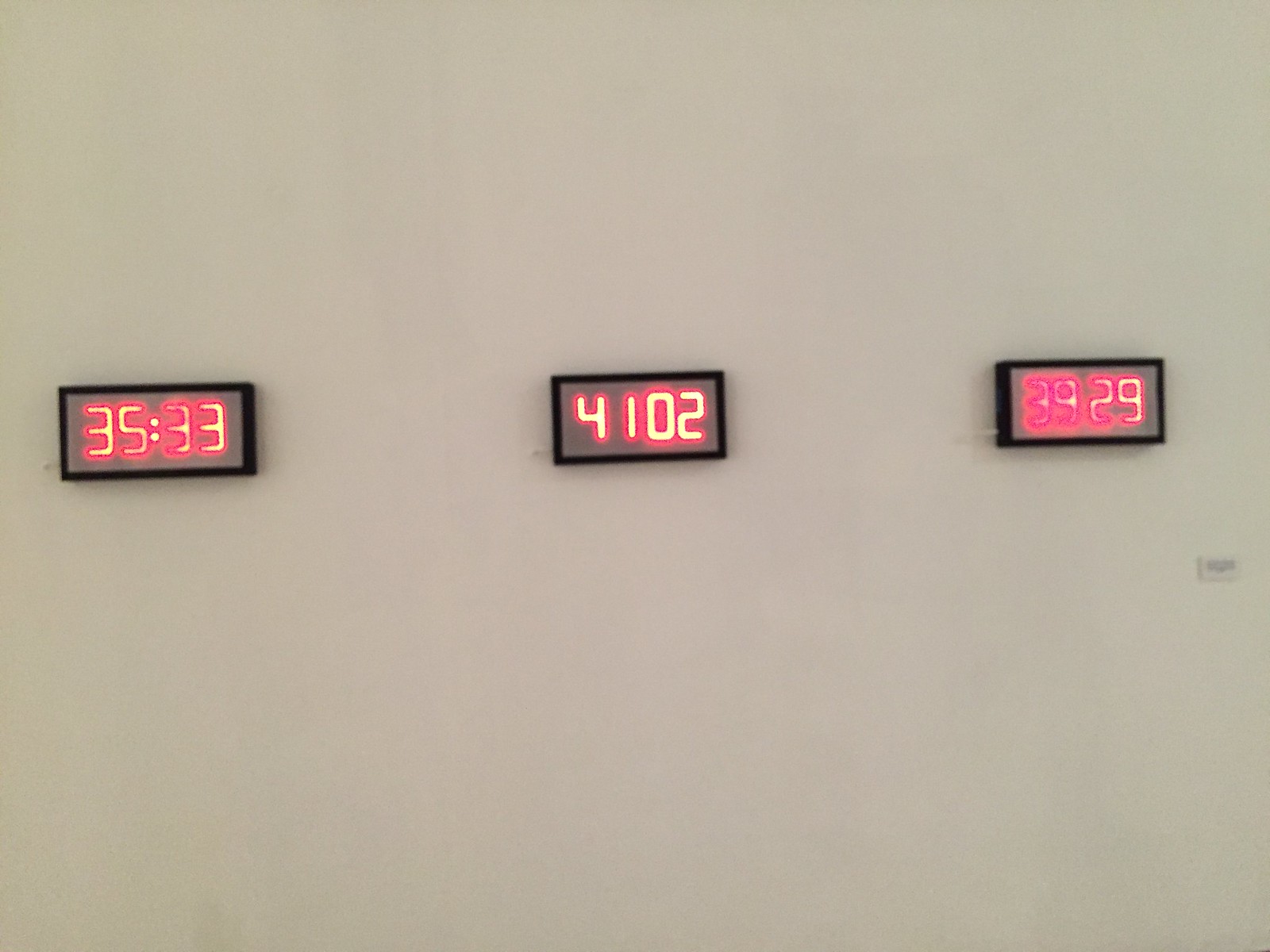This image captures a vibrant, possibly blurred color photograph or illustration, which may be intentionally designed to resemble a photograph. The focal point is an art installation mounted on a stark white wall, consisting of three square black-bordered rectangles evenly spaced in a horizontal line. Each rectangle contains a bright red neon number glowing vividly against the black background.

From left to right:
- The first rectangle displays the number "35:33," with a central yellow hue that enhances the glowing red outline.
- The middle rectangle features the number "4102," prominently illuminated in neon red.
- The rightmost rectangle presents "3929," glowing entirely in shades of red and pink with no yellow accent.

Beneath the right-hand rectangle, a small piece of paper is affixed to the wall, further suggesting this as an intentional art installation. The combination of neon colors and the precision of the arrangement creates a striking and modern visual impact.